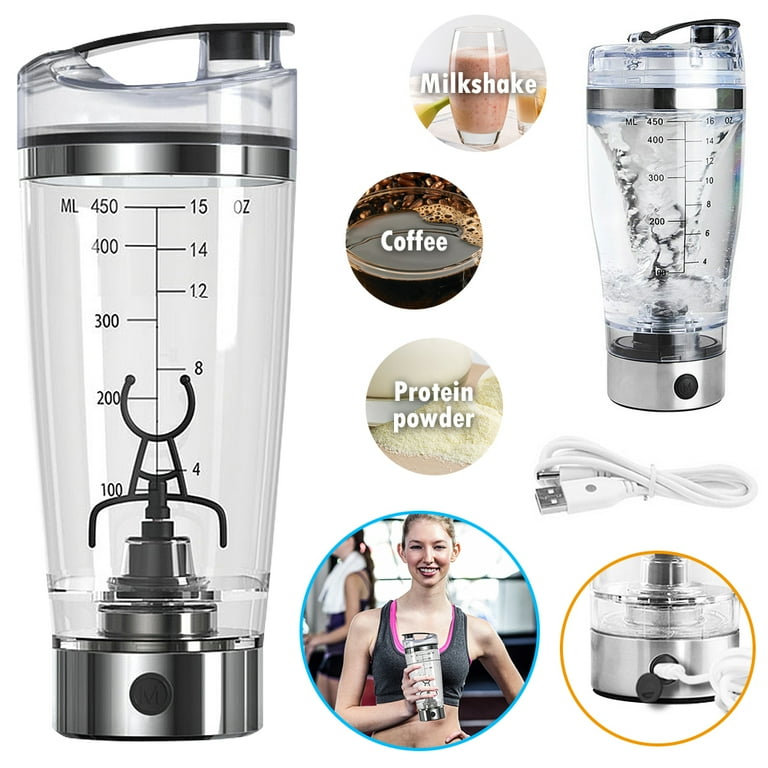This promotional image showcases a multifunctional, battery-operated handheld blender with a clear body, black internal components, and a silver base featuring a power button. The blender, shown upright on the left side of the image, has a screw-on cap with a gunmetal trim and a flip-top mouthpiece for drinking. Clearly marked with measuring lines, the blender is also depicted being held by a woman in exercise gear.

In the center, there are illustrative icons and labels denoting its versatile uses: "Milkshake" accompanied by an image of a pinkish-purple milkshake, "Coffee" indicated by a partial cup of black coffee, and "Protein Powder" represented by a pile of yellowish powder. A dynamic display on the right side shows the blender in action, creating a vortex in the liquid water inside. Below this, a white USB cord is displayed, showcasing the charging method for the blender. Overall, the image effectively highlights the blender’s various applications and practical design.